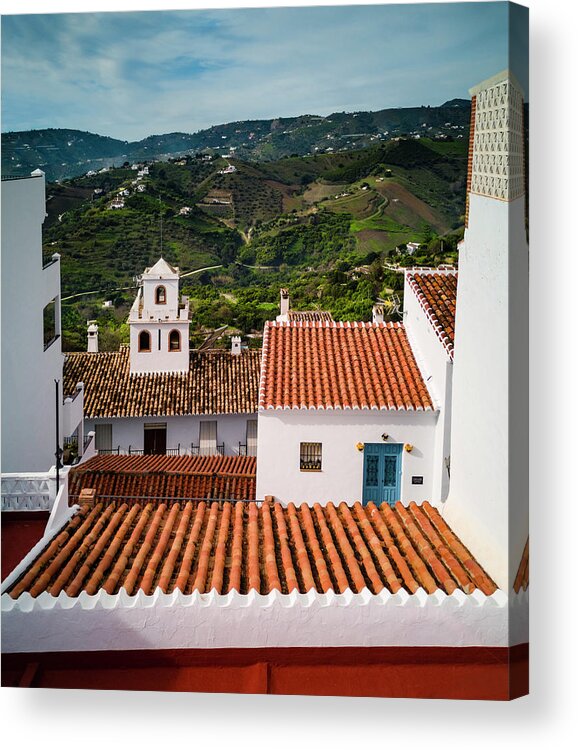The image captures a vibrant Spanish village, bathed in the warm light of a partly cloudy day. The top portion features a blue sky adorned with wispy white clouds that drift lazily across it. Below the sky, the landscape transitions into a series of green valleys and small mountains, their hues ranging from dark green to lighter shades interspersed with dense trees and foliage.

Scattered throughout this lush landscape are white houses with traditional terracotta roofs, creating a picturesque scene of serene rural life. The village stretches out with its network of dirt paths and winding roads, connecting homes and farmlands.

In the foreground, there is a prominent brown-roofed white house with a distinctive blue door. This house stands out, drawing attention with its rustic charm and terracotta tiles, framed by a white barrier around the roof's edge. Adjacent to this house is another white structure with a similar terracotta roof. Behind these, a taller building, possibly a church or bell tower, rises into view, its steeple adding to the village's timeless aesthetic.

Overall, the image, rendered on a stretched canvas, offers a bird's eye view of this quaint village, highlighting its harmonious blend of natural beauty and traditional architecture.